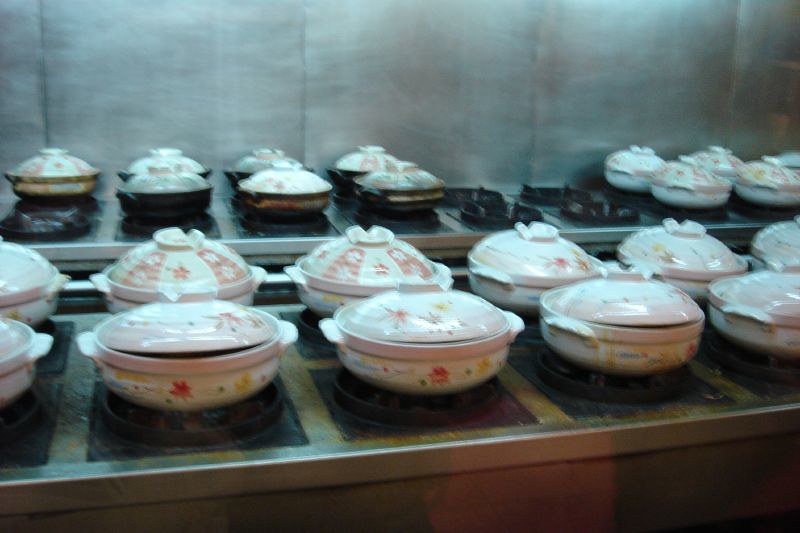This detailed photograph captures a bustling commercial kitchen with a long stainless steel stove cooking area. The stove is equipped with dozens of burners, almost all of which are occupied by about 20 low, round, white ceramic pots. These pots, featuring two distinct designs of pink flowers and stripes with flowers, come with lids and side handles. The scene shows four rows of these pots, some of which have brown liquid overflowing from the sides. The forefront of the image reveals a row of pots on a stovetop surface with hints of yellow and green coloring, while a further array of grills and pots extends into the background, set against a plain gray stainless steel wall. The entire area is well-lit from above, highlighting the industrious atmosphere as food is prepared in large quantities.